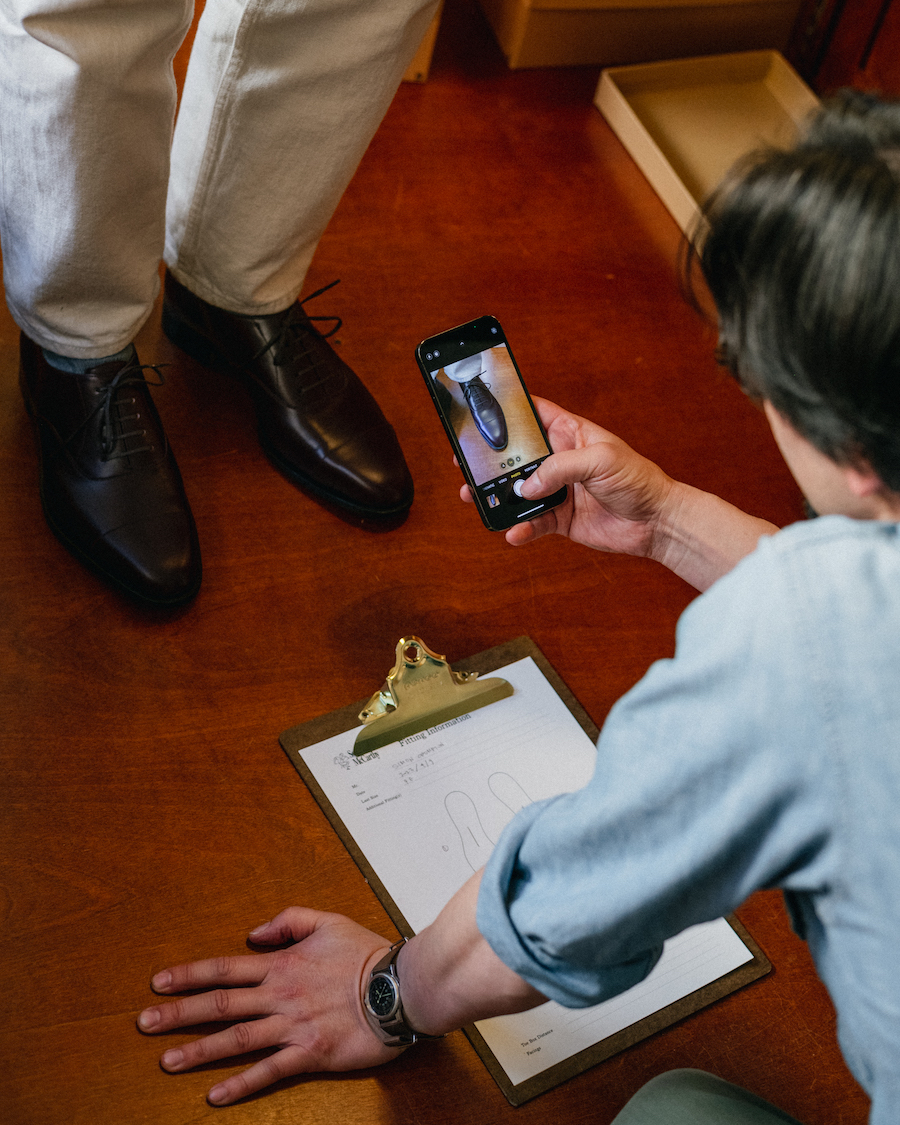The image depicts a scene with two men focused on a pair of shoes. A man with shiny brown shoes stands on reddish-brown hardwood floors. He is wearing light-colored jeans. In front of him kneels another man with shiny black, short hair, wearing a blue shirt with rolled-up sleeves, and a wristwatch with a brown leather strap on his left wrist. This kneeling man is using his right hand to take a photo of the shoes with his smartphone, while his left hand braces against the floor. On the screen of the phone, a close-up of one of the brown shoes is visible. Beside him on the floor lies a dark brown wooden clipboard holding a white piece of paper, possibly with a foot drawing and some text lines. Additionally, there are some boxes visible in the corner of the image, hinting at a setting focused on shoes or fitting, possibly indicating a shoe salesman or tailor at work.